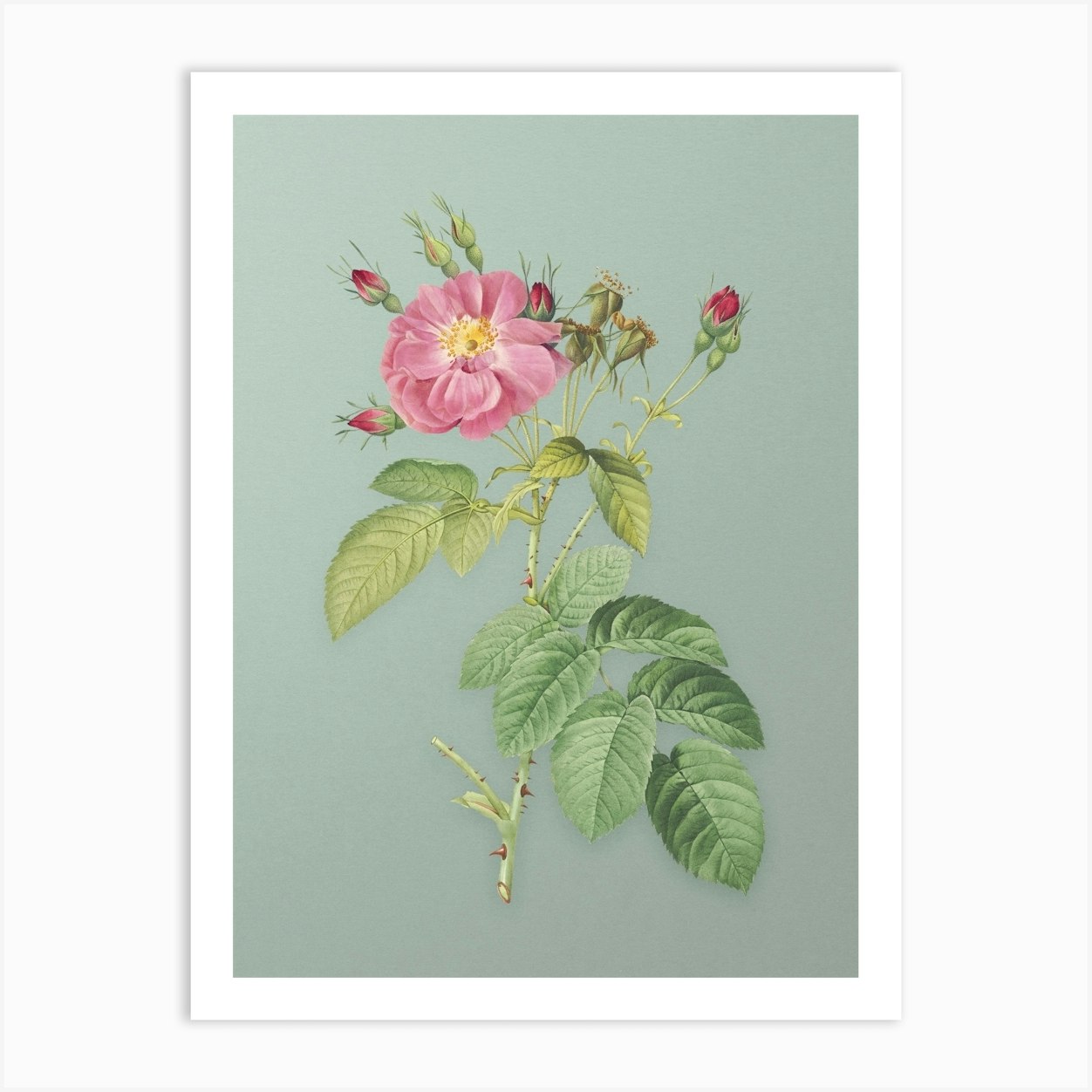The image is a detailed drawing of a flower, presented within a white frame that casts a drop shadow, suggesting it is mounted on a wall. The background of the artwork is a very light grayish teal color. The central focus is a large pink flower with light pink petals and a yellow center, which is depicted in full bloom. Surrounding the main blossom are several smaller buds, tinged with purple at their tips, poised to bloom. The flower’s stem, colored green with brown thorns, supports about five or six green leaves, especially noticeable at the bottom. This intricate botanical illustration seems to be rendered with colored pencils, giving it a soft and delicate appearance, much like one might find in a book or magazine.